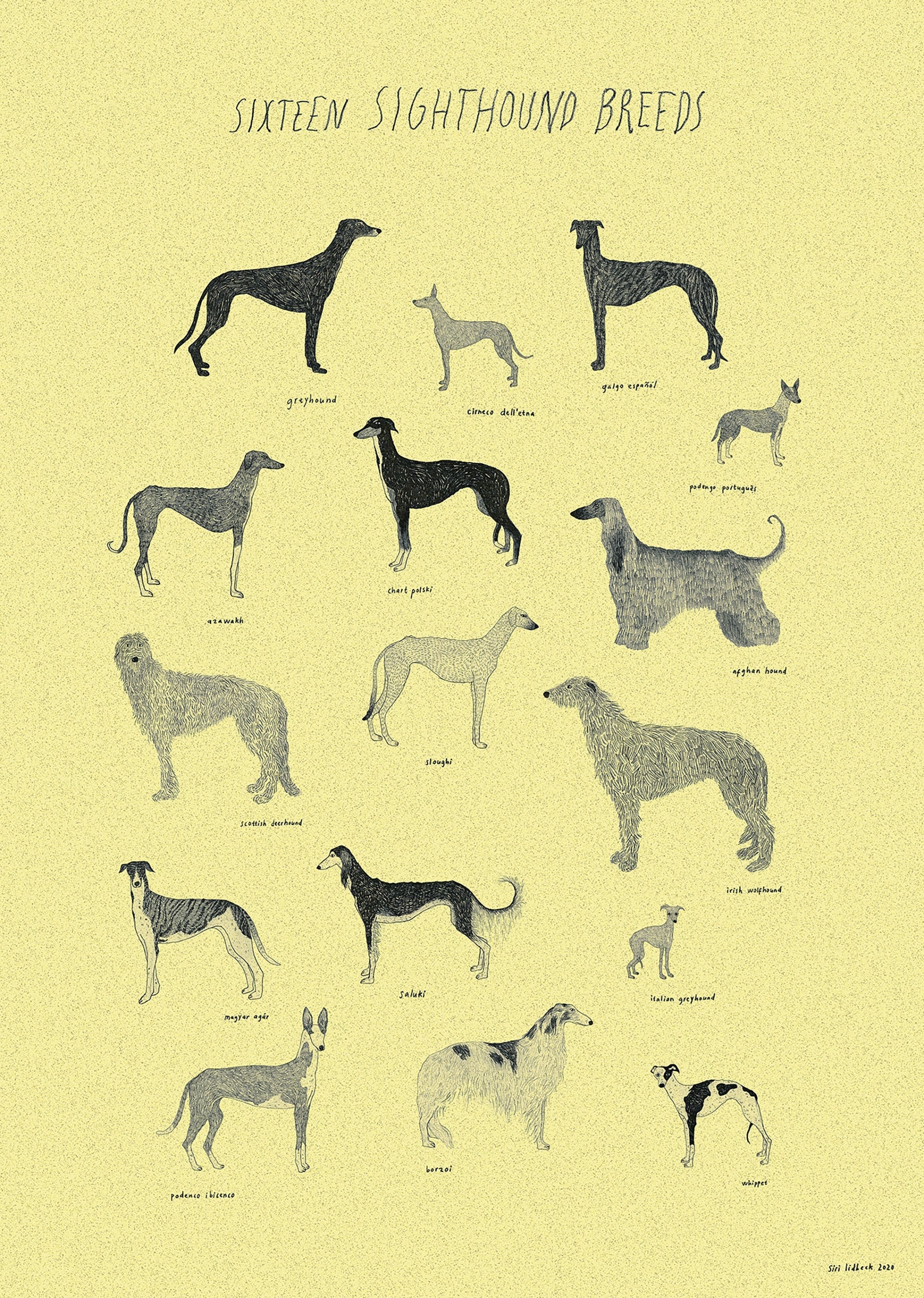The image appears to be a detailed poster, likely found in a doctor's office or educational book, with a yellow grainy background. At the top, in black lettering, it reads "16 Sighthound Breeds" in a slightly shaky font. Below this title, the poster features 16 black and white pencil drawings of various sighthound breeds, arranged in rows of three or four dogs per line. Each dog is depicted in a side profile and is intricately shaded to highlight their unique features. Beneath each drawing, the name of the breed is labeled in small black letters, although some of these names are difficult to read due to their size. Identifiable breeds include Greyhound, Galgo Español, Afghan Hound, Scottish Deerhound, German Sighthound, Irish Wolfhound, Italian Greyhound, Saluki, Magyar Agar, Podenco Ibicenco, Borzoi, and Whippet. This poster was created by Siri Lidbeck in 2020.